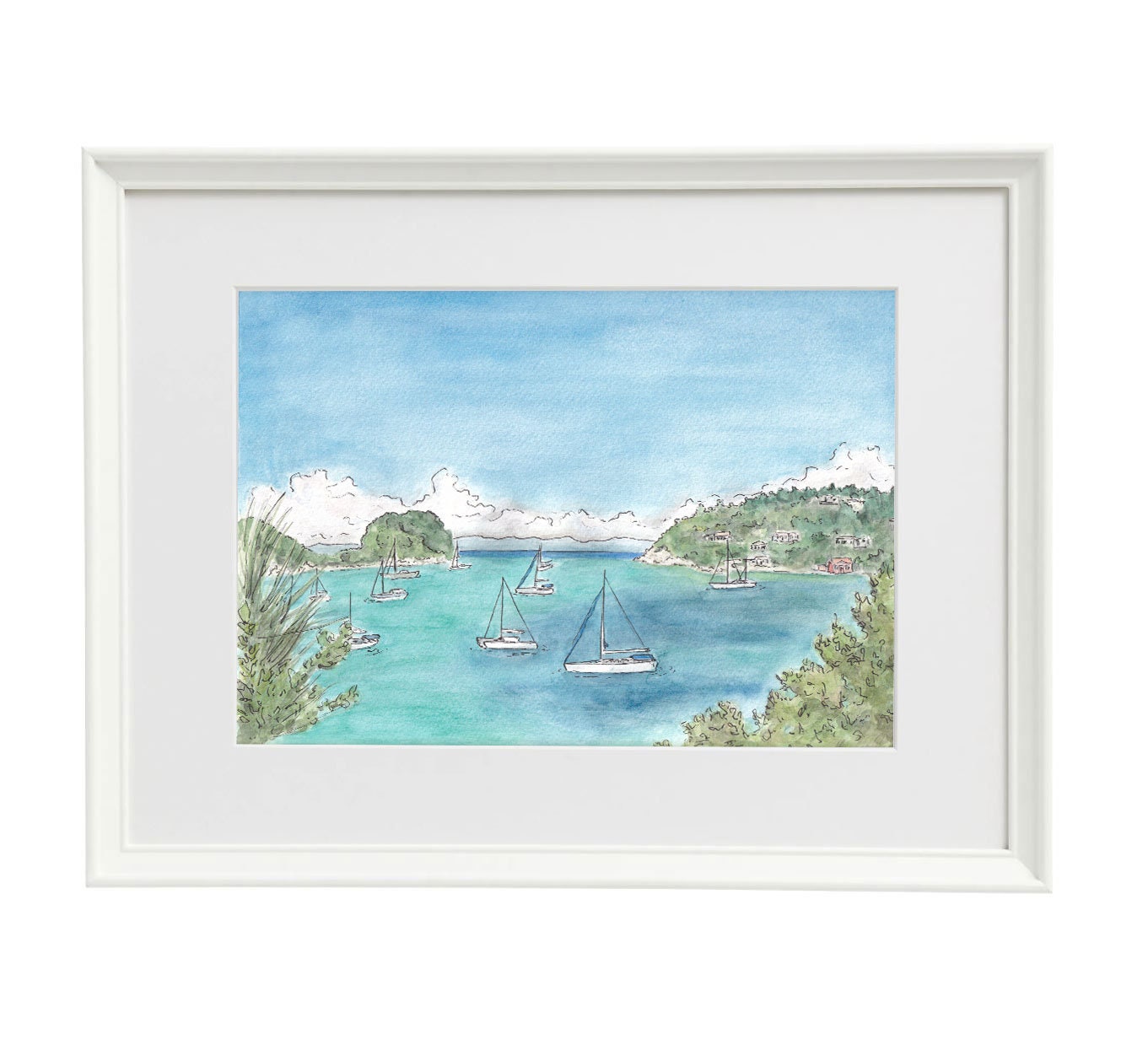This is a framed watercolor and pen-and-ink painting depicting a serene ocean harbor scene. The artwork, enclosed in a white wood frame with a white mat, features an array of ten sailboats scattered across varying shades of blue water, transitioning from light turquoise to deep navy as the sea deepens. The boats, with their white bodies and translucent sails, allow glimpses of the water through them. Surrounding the harbor are verdant green trees and hills, giving the impression of a remote, natural setting. In the background, there's a patch of low-lying land and clusters of small houses nestled on the hillside. Above the harbor, a gradient sky transitions from light to dark blue, dotted with white, puffy clouds that stretch across the scene, enhancing the tranquil atmosphere.